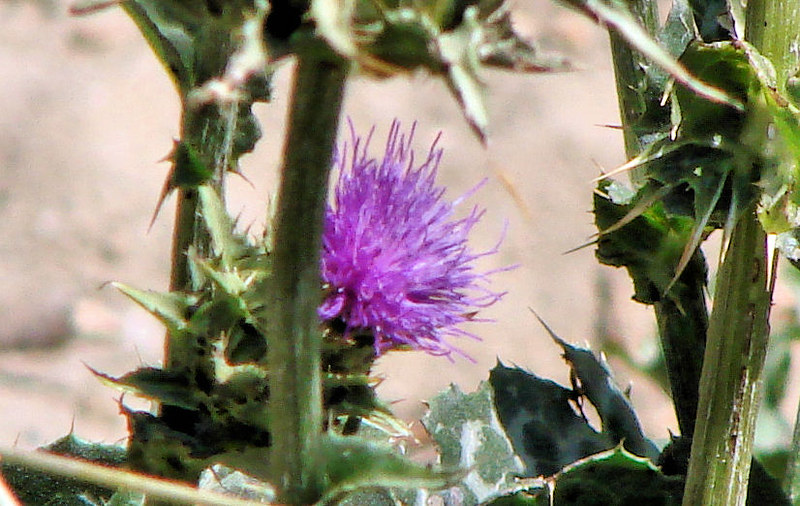The image depicts a robust plant reminiscent of a milk thistle or a similar species, characterized by its vivid purple, spiked flower that resembles a pom-pom or clover bloom with thin, antenna-like strands fanning out. The flower is surrounded by coarse green stems and leaves, all of which are adorned with sharp, spiny thorns, adding a defensive, prickly texture. The dense, ribbed stems provide a solid structure to the plant. In the background, there is a blurred, rough-textured tan area, possibly a rock or dirt hill, indicating the plant is thriving in an outdoor, sunlit, somewhat barren environment. Some leaves appear to have been nibbled, hinting at interactions with small wildlife.